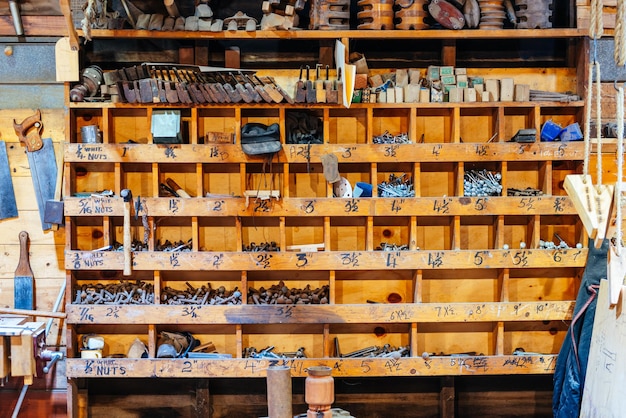This detailed image captures the essence of a busy carpenter's workshop. At the center is a large, honey-colored wooden organizing system, featuring five rows of compartments that house a variety of hardware such as screws, bolts, and nuts. The top three rows contain smaller compartments, while the lower rows accommodate larger ones. Each compartment is meticulously hand-labeled with measurements, denoting the increasing sizes from left to right.

Hanging prominently on the left wooden wall are two saws, with a vise positioned underneath them. Adjacent to these tools is an item that appears to be a solid, indistinguishable object, possibly a paintbrush or another tool. The scene further reveals a workbench equipped with a wooden vise for holding projects in progress.

On the top shelf of the organizing system, and across the top row, there are various difficult-to-see objects, including block and tackle units. To the right side of the image, one can identify a blue apron hanging alongside other tools wrapped in a tarp. The overall setup, though it may seem messy at a glance, is highly functional, indicating a workspace that is regularly used. The carpenter’s tools are well-organized, with nuts labeled in predefined measurements, evidencing systematic usage in everyday tasks.